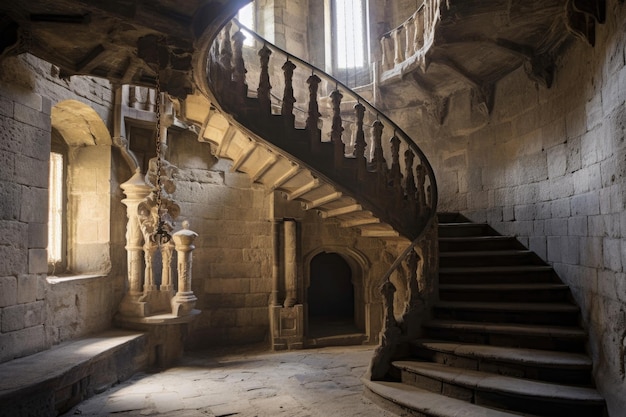The image depicts a grand, old-style castle interior characterized by a spiral staircase constructed mainly from concrete. The staircase elegantly coils upward from the right side of the picture to the left, leading to a rounded upper level that features a balcony attached to the building's right wall. The walls are composed of cinder blocks, adding to the rustic feel of the scene, which is bathed in natural light filtering through an R-shaped window on the left. This window, with its golden-hued light, includes a step-up section with a built-in seating area beneath it and is flanked by a couple of posts. Below the window, there's a little archway, shrouded in darkness, possibly leading to a hidden storage space. To the right of the picture, additional light streams from an unseen source, illuminating parts of what appears to be a historical setting, complete with statue-like figures resembling chess pieces, adding to the regal and somewhat mysterious ambiance.